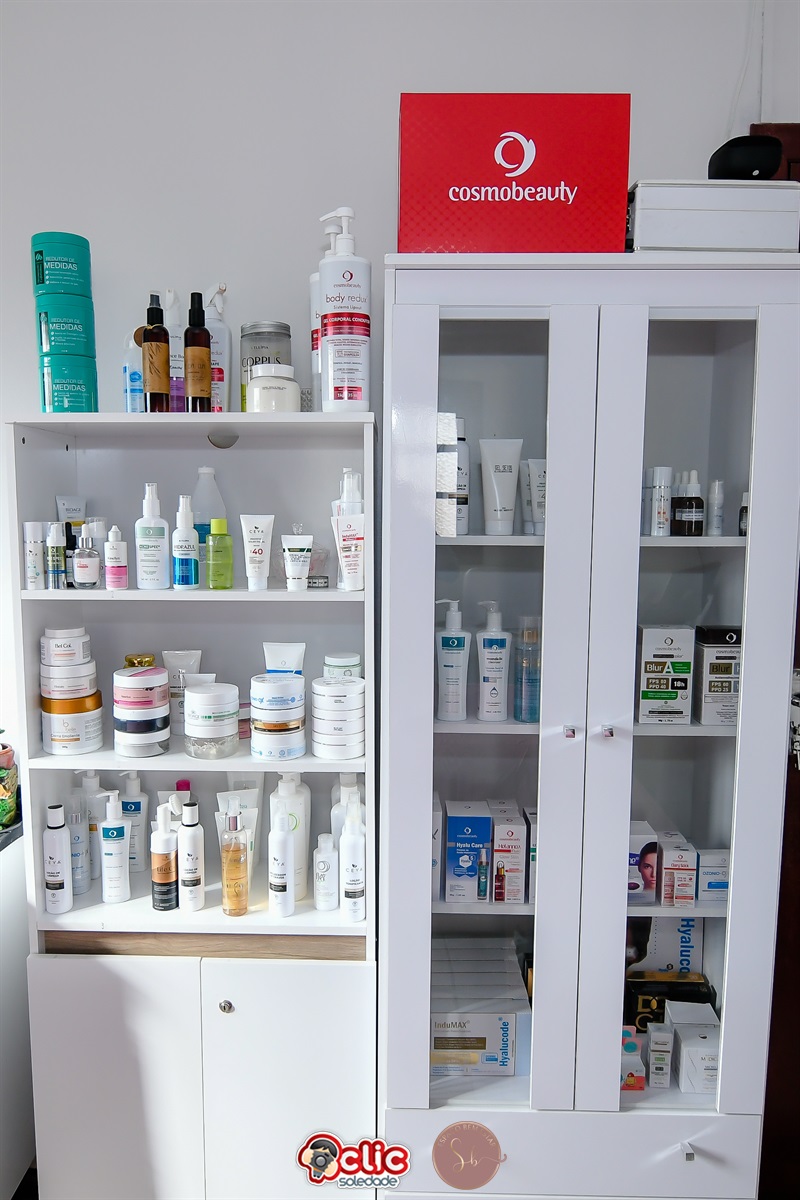The photograph showcases a well-organized display of various beauty products arranged on shelves. On the left, there is a shelving unit with double doors at the bottom and four open, bookcase-style shelves above, filled with an array of items. To its immediate right is a white bookcase with four shelves, completely enclosed by glass-panelled doors, allowing visibility of the contents within. This white bookcase also features a single drawer at the bottom, equipped with two sleek drawer pulls. Atop this white unit is a prominent red rectangular sign with white text reading "Cosmo Beauty," accompanied by a circular logo. The shelves are stocked with a diverse assortment of beauty products, including pump bottles, round-lidded containers, lotion bottles, and various boxed items, each carefully arranged to attract attention.